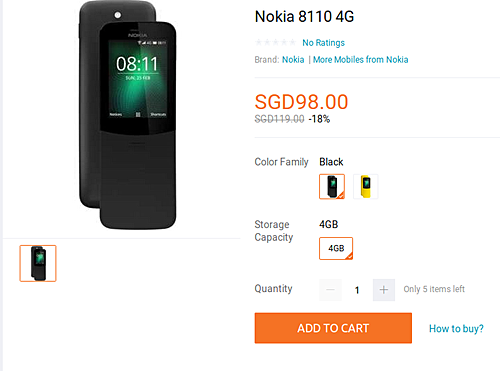This image showcases the Nokia 8110 4G, a model that evokes a sense of nostalgia with its primitive and minimalistic design. Displayed on a retail page, the phone's specifications and purchase options are highlighted in various sections of the image. The top part of the phone prominently displays the iconic Nokia logo, which is a clickable hyperlink taking you to Nokia's main page, with another separate hyperlink offering more mobile options from Nokia.

Originally priced at SGD 119.00, the Nokia 8110 4G is now available for SGD 98.00, reflecting an 18% discount. The phone comes in two color variants: currently highlighted is the black version, but a yellow option is also available. The only storage capacity listed is 4G. There’s an indicator showing a limited stock with only five units left, and an option to add the desired quantity to the cart is provided. Adjacent to this is another hyperlink explaining "how to buy."

The product images display both the front and the back of the phone. The Nokia 8110 4G deviates from the contemporary smartphone look, featuring a long, solid design without a flip mechanism. The top half of the phone incorporates the screen, which appears to be touch-capable, displaying the interface with battery life, signal strength, time (8:11), and a green spiral wallpaper. The bottom half remains a solid black, devoid of any screen space. Additionally, there’s a depiction of the phone in its slide-open state.

In the bottom left corner, a smaller, minimized version of the same detailed image provides an additional perspective. The phone’s basic and unadorned style suggests it might be catering to a different market or user preference, emphasizing simplicity and functionality.